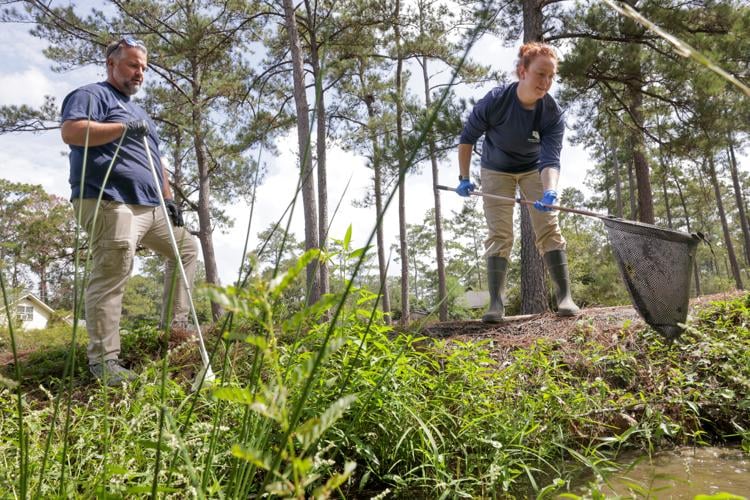In a sunlit outdoor setting, a red-haired woman and a man, both in blue t-shirts with matching khaki pants and boots, are engaged in what appears to be a form of collection work or environmental research. They stand near a small, brackish pond, surrounded by slender trees and tufty green grasses. The sky above is a mix of blue and white clouds, casting a bright but dappled light on the scene. The woman, whose hair is tied into a bun, is intently using a large net, almost knee-deep in rubber boots, seemingly catching or retrieving something from the water's edge. The man, holding a white pole, watches her closely. Both are focused on the task at hand, suggesting a sense of purpose, whether scientific or environmental. The tranquil environment, with its sparse trees and patches of greenery, adds to the intricate detail of their activity, encapsulating a moment of concentrated effort in nature.